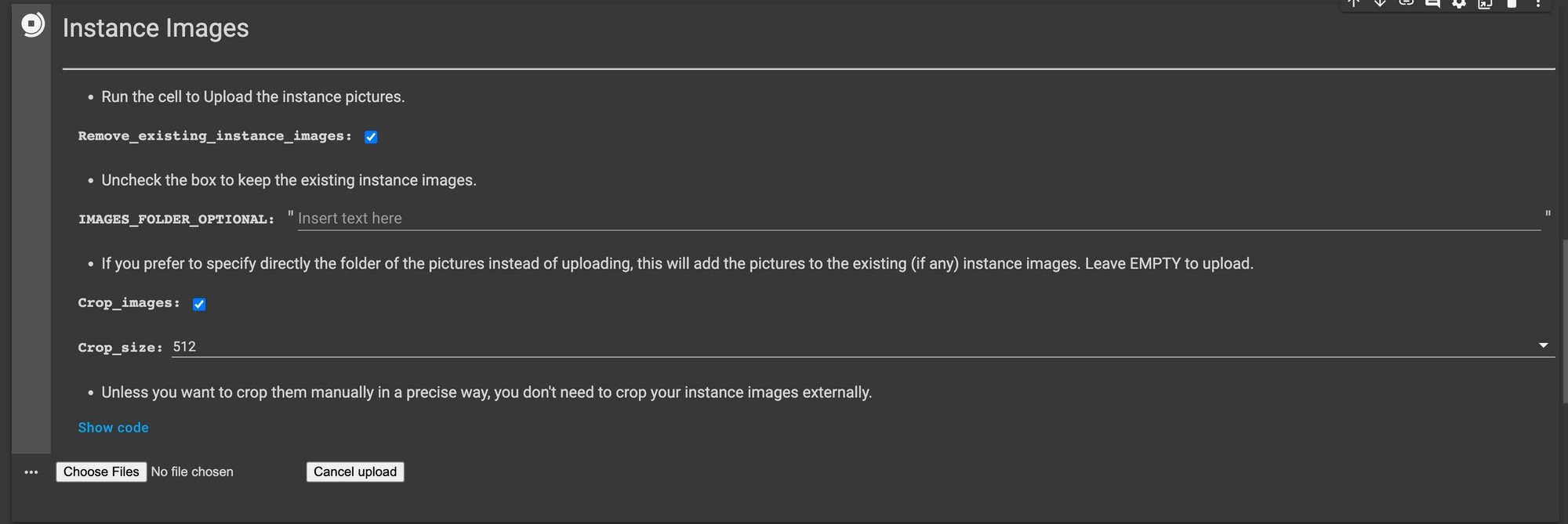The screenshot features a predominantly black screen with light gray text. The text provides instructions and options for managing images within a system. Specifically, it reads:

- "Instant images: Run the cell to upload instant pictures."
- "Unlock the box to keep the existing instant images."
- "If you prefer to directly order upload photos instead of uploading, they will add the pictures to the existing instant images. Leave empty to upload crop images."

Additionally, there are interactive elements including checkboxes and buttons:
- A checkbox marked "Crop images" is selected.
- A checkbox marked "Remove existing ones" is also selected.
- A blue button labeled "Show code."
- "Choose files" and "Cancel upload" buttons for file management tasks.

Overall, the interface appears to give users control over uploading, cropping, and preserving or replacing existing images with new ones. The detailed options and instructions suggest a focus on customizable image upload and management processes.